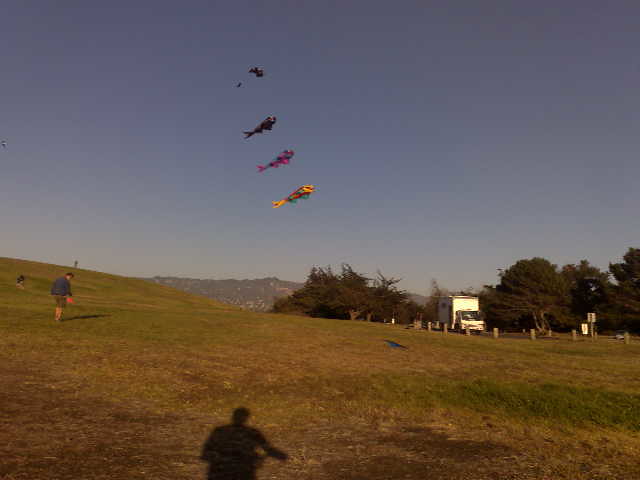In this photograph, a sprawling, grassy hillside stretches into the distance, slightly out of focus, framed by a serene, grayish-blue sky. At the far end of the field, a solitary man in a green jacket and brown shorts stands out prominently, holding an orange kite reel, while another man’s shadow can be seen in the foreground, suggesting he too is engaged in the activity. The scene is dotted with vibrant person-shaped and fish-shaped kites in the air, boasting hues of yellow, red, pink, orange, teal, and blue, some forming complex shapes high above. The ground below mirrors this aerial spectacle with shadowy kite silhouettes. A large white delivery truck is parked near a less-traveled road lined with wooden posts. Behind this, amid a sparse parking area, trees and distant mountains provide a majestic backdrop, emphasizing the expansive and tranquil nature of this kite-flying haven.